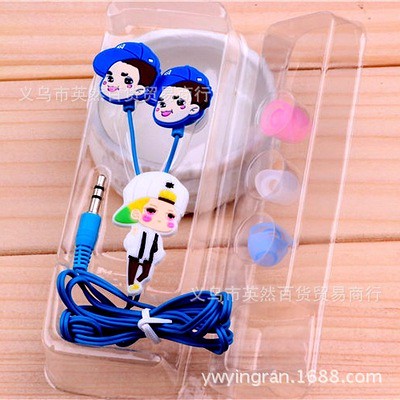The product image showcases a wired headphone set encased in clear plastic packaging. The blue earbuds feature an anime-like design with characters on each earpiece; these characters wear blue hats, have brown hair, white faces, and big smiles with circles on their cheeks. On the back side of the earbuds, there is a detailed image of a boy wearing a white baseball cap backwards, with pink cheeks, a white coat, black pants, and yellow shoes. At the junction where the two cords merge, another full-body image of the boy can be seen. The cords are predominantly blue and still wrapped within the plastic case. Additionally, the packaging features extra earbud cushions in pink, white, and blue. There is also a website displayed in the bottom right corner, reading YWINGRAN.1688.com. Chinese or Japanese writing appears along the photograph in white.